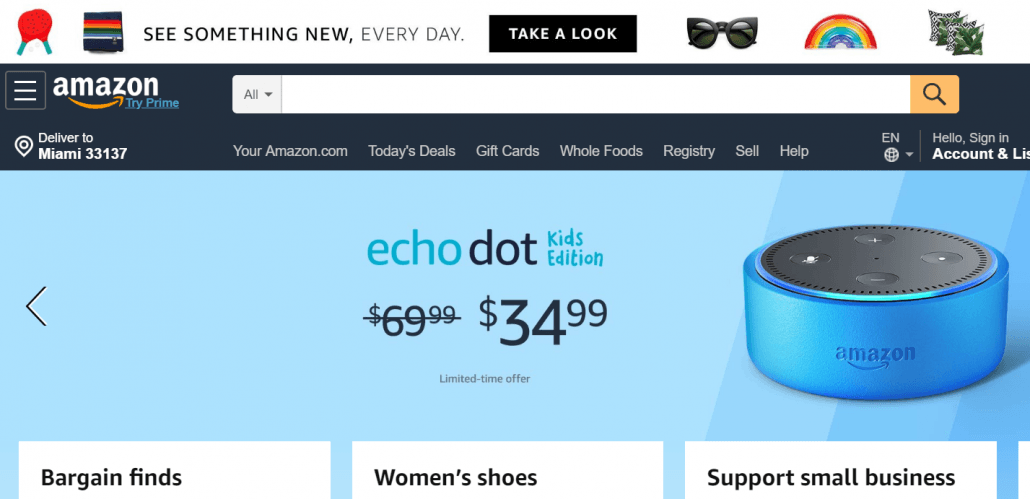The image depicts the Amazon website's homepage with several elements clearly visible. On the upper left-hand side, the Amazon logo is prominently displayed. Below it, a grayish bar stretches horizontally across the page, featuring an advertisement for ping pong paddles.

Beneath this grayish bar, there is another product image that appears to be a black, red, and white square item. Accompanying this is a tagline that reads "See something new every day", positioned prominently in the center above a black button with white text that invites users to "Take a look".

Further down, another set of product images includes sunglasses, a rainbow-colored item, and what appears to be a tree-themed item. Below these images lies the Amazon search bar. Just beneath the search bar, the delivery location is specified as "Deliver to Miami 33137".

The navigation menu is visible and includes links to various sections such as Youramazon.com, Today’s Deals, Gift Cards, Whole Foods, Registry, Sell, and Help. The language is set to English, and there's a prompt for users to "Hello, Sign in". Additionally, the banner prominently features an Echo Dot product advertisement.